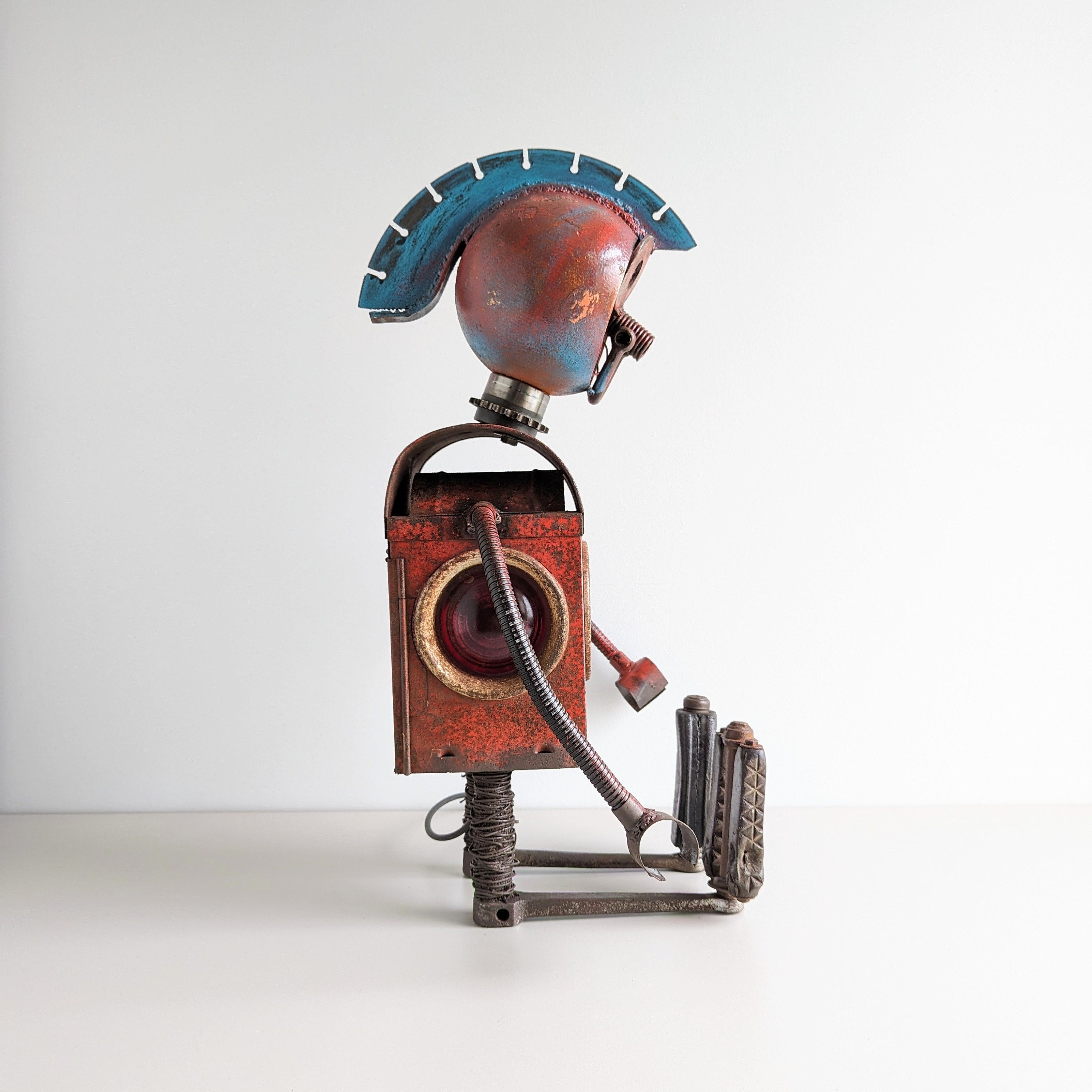The image features a detailed piece of metal art depicting a small robot-like statue seated on an off-white surface against a solid white, light-gray shadowed wall background. The robot is crafted from various pieces of metal machinery and equipment, giving it a distinct, warrior-like appearance. The head is a round knob resembling a shift gear, fitted with a screw for the nose and topped with a distinctive blue mohawk across its head. The neck appears to be made from a gear. The body is an orange, rusty-looking rectangular box with a large, camera-like lens or red jewel in the center. 

The legs, composed of thin metal bars wrapped in silver wire, are flat on the surface with the feet pointed upwards, featuring bolts at the tips. The knees are indicated by bicycle pedal arms, providing a recognizable bend. The arms extend from the body like thin, coiled wire resembling electrical wiring, ending in hooked, door-stopper-like hands or clamps. The overall composition of the robot reflects intricate detailing, robust construction, and a whimsical mix of industrial and artistic elements.